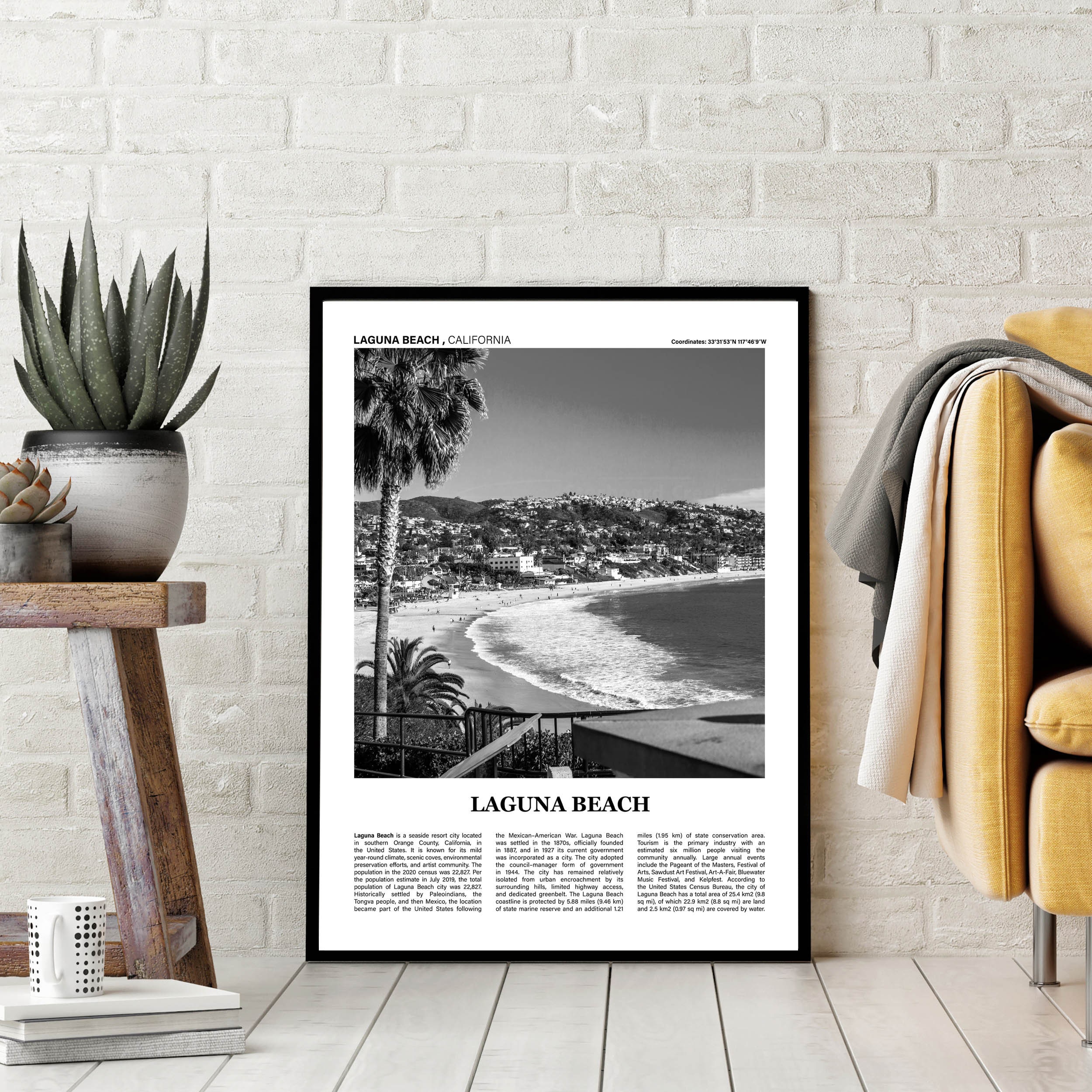The photo depicts a minimalist room with a white wooden floor and a white brick wall. Central to the image is a framed poster for Laguna Beach, California, featuring a large photo of the beach with buildings, hills, palm trees, and the ocean, as well as people enjoying the scenery. The poster includes black text at the top and the bottom, with "Laguna Beach" prominently displayed in large letters and several paragraphs of information beneath the photo, all encased in a black frame.

To the right side of the frame, a yellow chair or sofa is partially visible, with tan cushions and fabric draped over the armrest—dark gray and lighter-colored textiles hang over the edge. 

To the left side, there is a small wooden table holding a stack of canvases and a white mug with black spots. Two desert plants, possibly agaves, are potted nearby. The overall color scheme is light and airy, with muted tones dominating the scene.